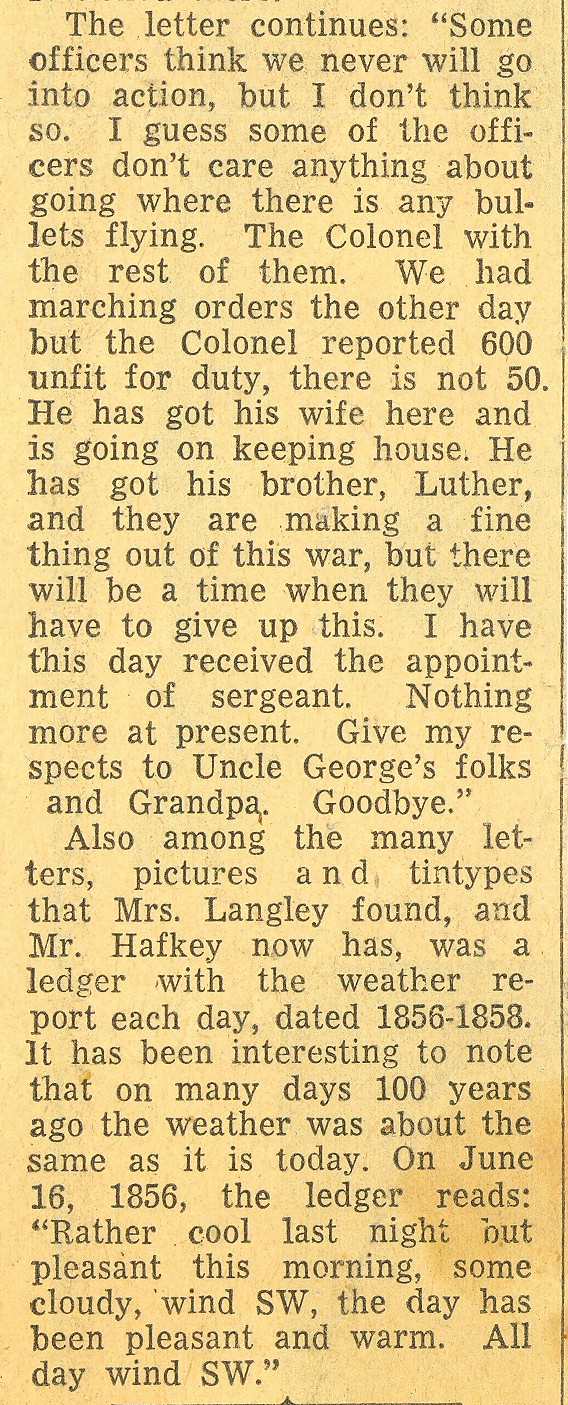This image is a yellowed newspaper clipping featuring black text, occupying a slender, rectangular column three times higher than it is wide. The clipping primarily contains two paragraphs from a historical letter discussing experiences during a war. The letter begins with the continuation, "Some officers think we never will go into action, but I don't think so. I guess some of the officers don't care anything about going where there are bullets flying." The writer critiques their colonel, who reported 600 soldiers as unfit for duty despite, in the writer's opinion, there being fewer than 50. The colonel, his wife, and his brother Luther, who are profiting from the war, are also mentioned. The letter notes, "I have this day received the appointment of sergeant," and ends with, "Give my respect to Uncle George's folks and Grandpa, goodbye." Additionally, the clipping includes a section about various items discovered, such as a weather ledger from 1856-1858, which intriguingly reveals similar weather patterns to those of today. On June 16, 1856, for instance, the ledger recorded, "Rather cool last night but pleasant this morning. Some cloudy winds southwest, the day has been pleasant and warm all day, winds southwest."